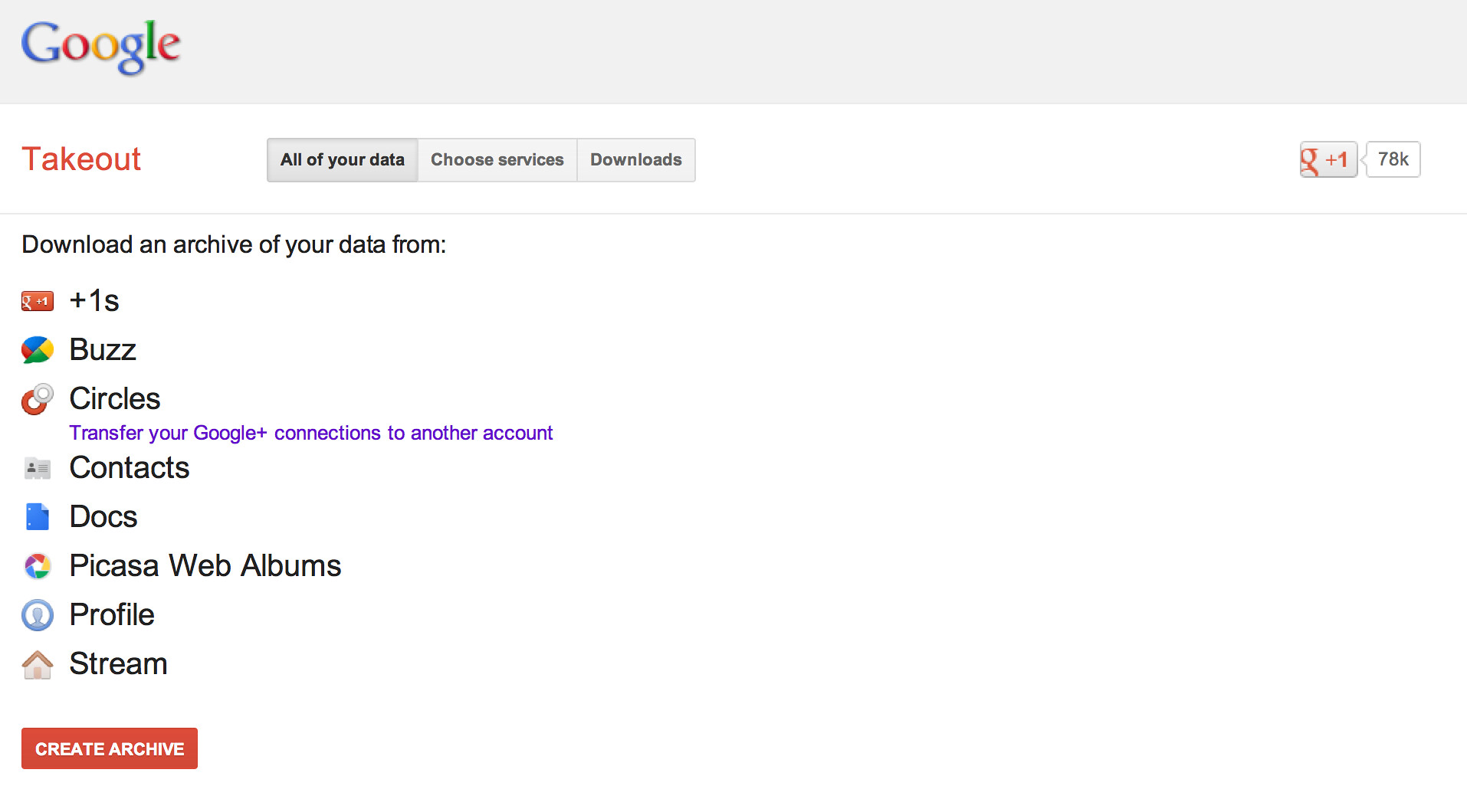The image displays a Google Takeout interface in detail. At the top, a light blue border stretches across the screen, and in the top right corner, the Google logo is prominently displayed with letters in specific colors: a blue "G," red "O," yellow "O," blue "G," green "L," and red "E." Below the border, the background is entirely white. Centrally, "Google Takeout" is written in a combination of white and red text.

Adjacent to the "Google Takeout" text, there are three horizontally aligned buttons labeled "All Your Data," "Choose Services," and "Downloads." On the far right side of the screen, there's a small button featuring a red "G" with a plus sign and "1" next to it, followed by a white square bearing "78K."

Under the "Takeout" heading, black lettering spells out "Download and archive from your data." Beneath this text is a brown emblem with the label "+1s" beside it. To its right is a multi-colored chat button—blue on top, yellow on the right, green at the bottom, and red on the left—next to the word "Buzz." Below this section, a large red circle overlaps a smaller white circle, emphasized by the label "Circles." Below "Circles," blue text advises, "Transfer your Google Plus connections to another account."

Further down, the interface displays various icons representing different Google services: a small white square with "Contacts" written to its right, a blue square followed by "Docs," a multi-colored circle (red at the top, yellow on the side, blue at the bottom, purple on the left) next to "Picasa Web Albums," and a white circle outlined in blue containing a person icon by the word "Profile." Below this, a tiny house icon is adjacent to the word "Stream."

At the bottom of the interface, a red rectangle with white lettering commands, "Create Archive."